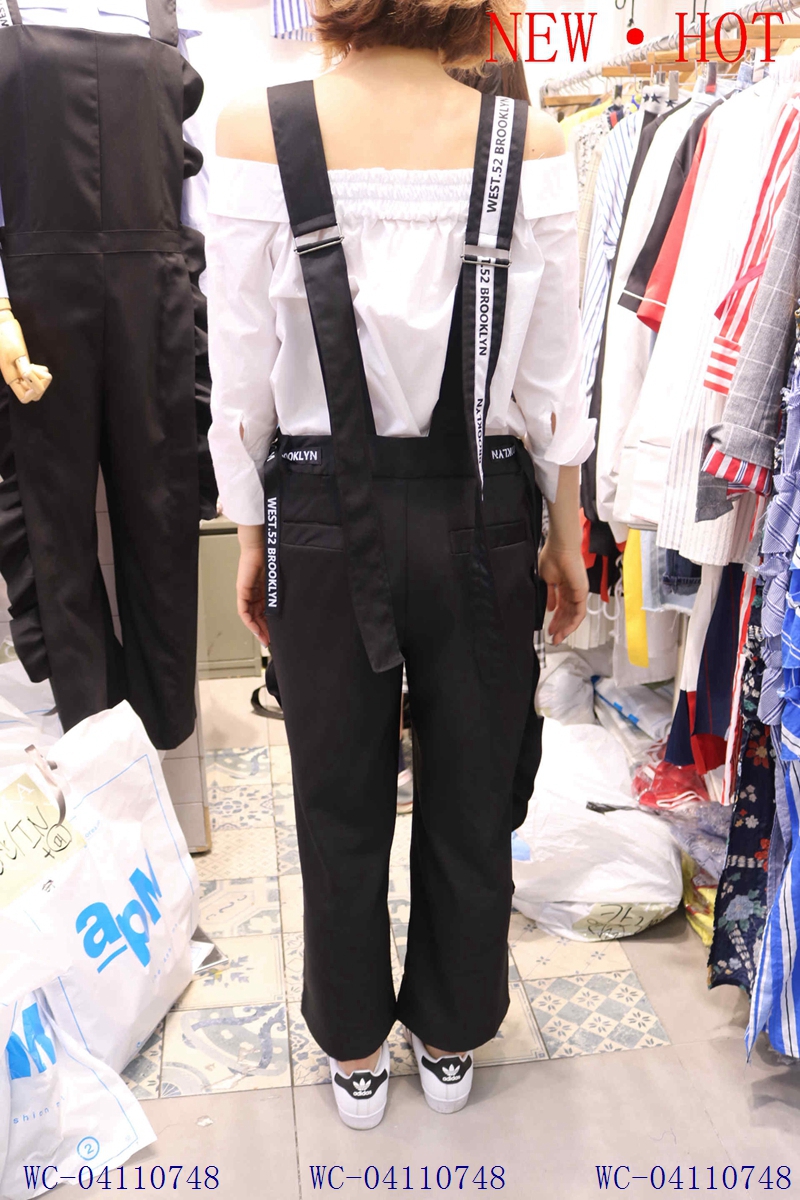The photograph captures the back of a light-skinned woman with short, round hair standing in a well-lit clothing store. She is wearing a white off-the-shoulder blouse that features frills along the back. Over her blouse, she has on black dress pants that come up to her waist, with black cloth suspenders featuring white stripes and the text "West.52, Brooklyn" running along them. Her white Adidas sneakers have black tabs and a clover-like symbol. To her left, there are two white shopping bags with blue "APM" lettering, while a mannequin dressed in matching black pants and suspenders stands on her left. To her right, there are racks filled with clothes. At the top right corner of the image, red block letters spell out "NEW.HOT," and at the bottom of the picture, in dark blue text, the catalog number "WC-04110748" is repeated three times. She is standing on a gray tiled floor accented with a multi-patterned white and blue rug.